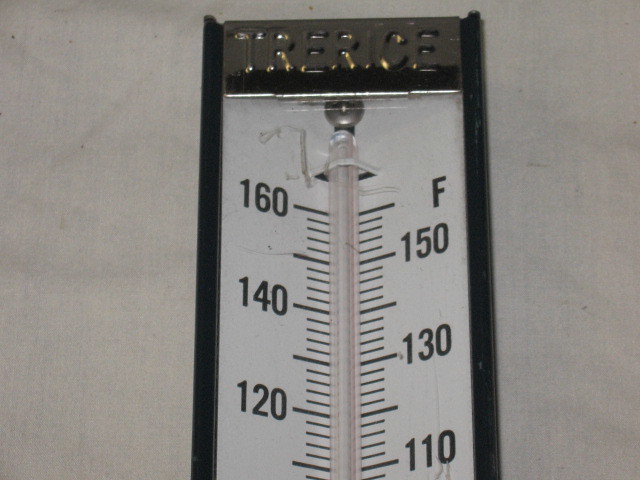This photograph features a temperature gauge placed against a white muslin fabric background. The fabric is noticeably marred with light gray marks and some wrinkles, especially concentrated in the upper left corner. While not filthy, the fabric is clearly used and imperfect. The temperature gauge itself reveals partial numerical readings, starting from 110°F at the bottom right and ascending in increments up to 150°F, with the scale labeled in Fahrenheit. On the left side of the gauge, the numbers progress from 120°F to 160°F, with horizontal black lines demarcating each temperature level. The red temperature indicator is absent, suggesting the detected temperature is below 110°F. At the top of the gauge, there is a metallic logo displaying the brand name "Trerice."